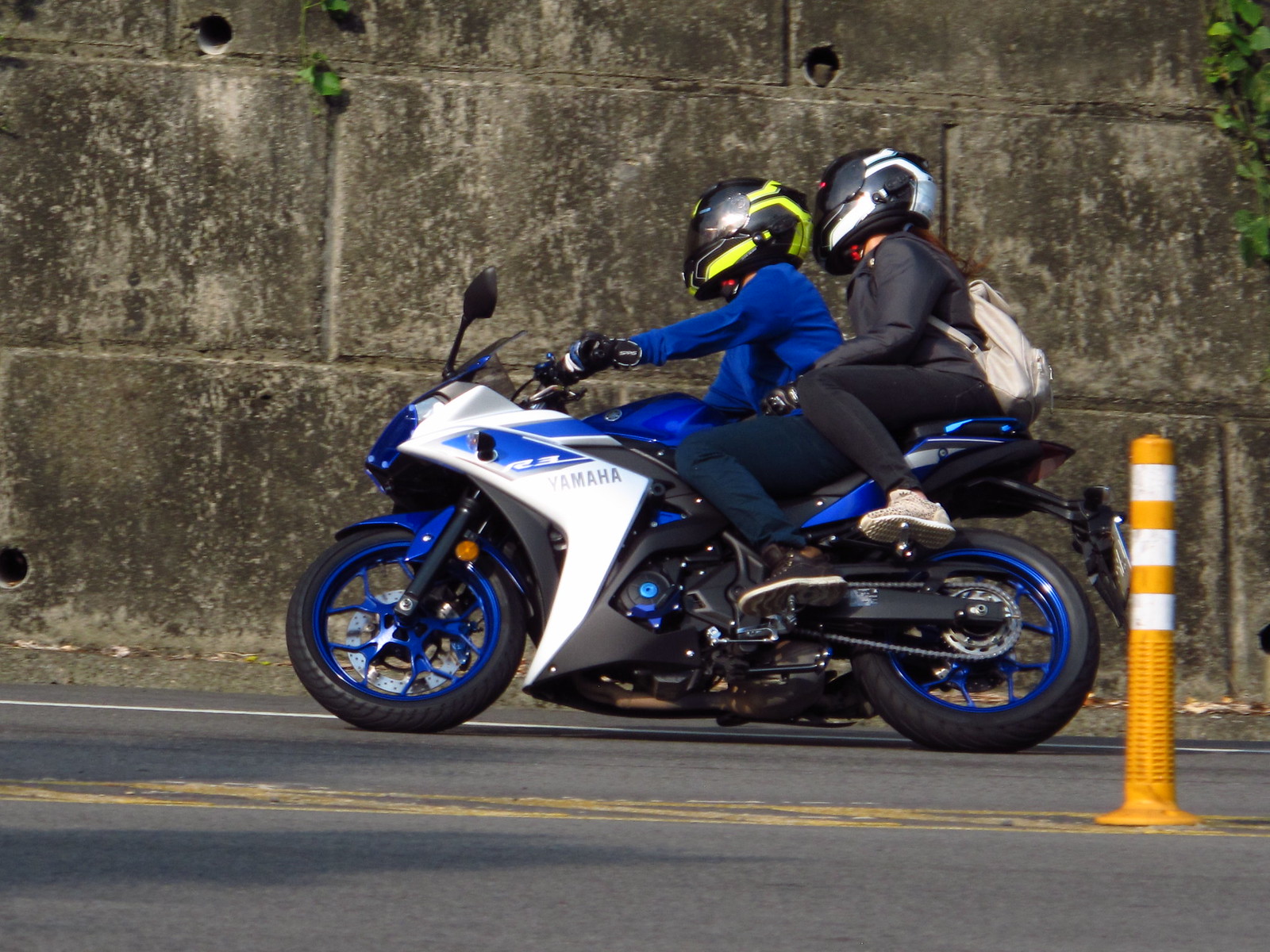This full-color outdoor photograph, taken during the daytime, features a couple riding a white and blue Yamaha motorcycle on a paved road. The motorcycle has blue rims and some black details. The driver, portrayed in profile as the bike moves left, wears a blue long-sleeve shirt, dark blue pants, dark sneakers, and gloves, along with a black helmet with yellow and chartreuse accents. The passenger, sitting behind and holding the driver's waist, dons a black jacket, black leggings, and light-colored tennis shoes. They also wear a black and white helmet, and carry a white backpack; their long hair is visible from the back of the helmet. The setting includes visible yellow median lines and an orange cylindrical barrel with white stripes, situated on the right side of the road. A significant retaining wall made of large, possibly brownish-gray or gray cinder blocks with drainage holes provides a backdrop to the scene.